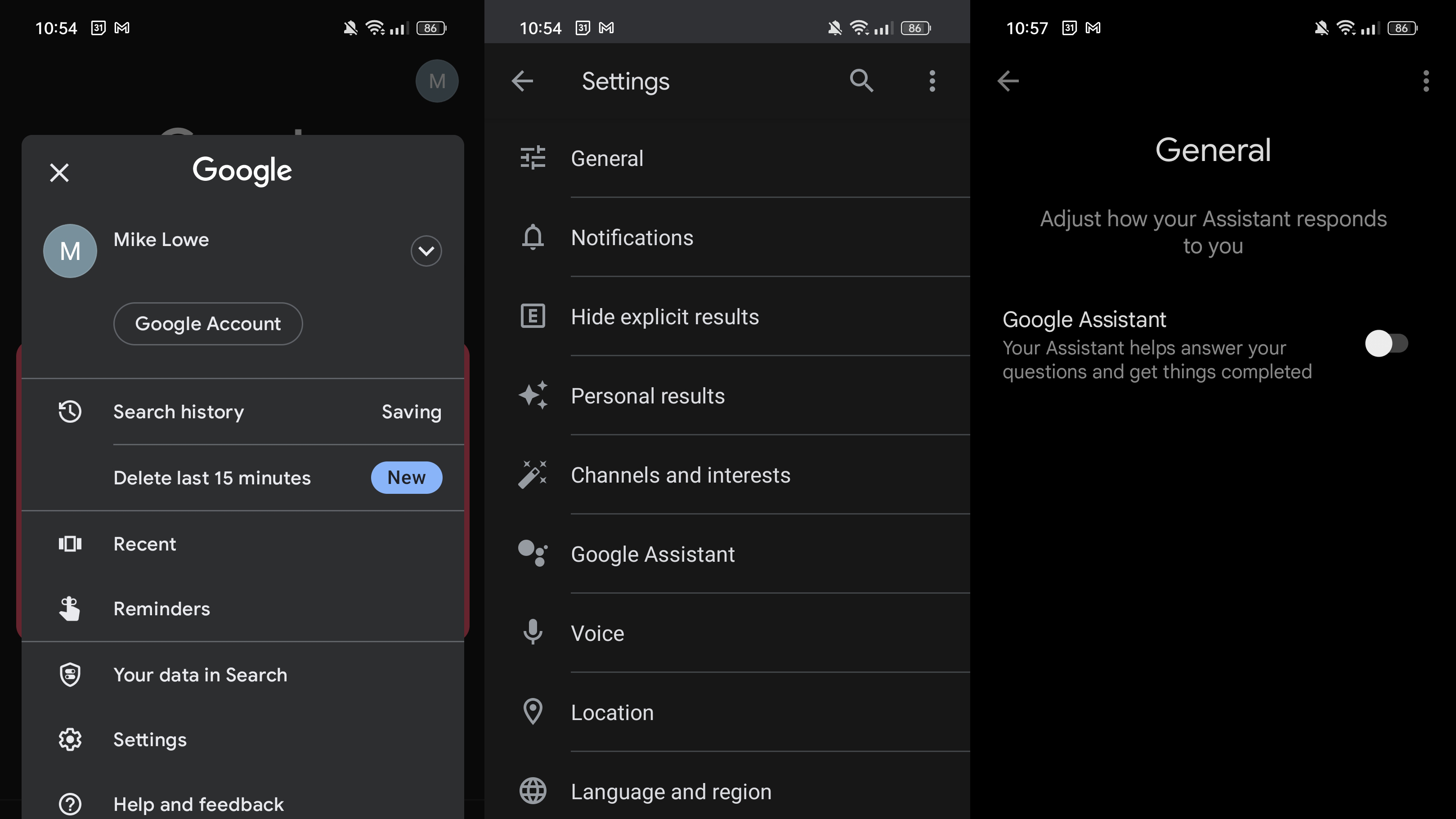The image is a composite of three screenshots from a mobile device, each showcasing different settings and options. Here's a detailed caption:

---

**A Composite Image of Mobile Device Screenshots Displaying Google Account Settings and Features**

**Left Screen:**
- **Background:** Black
- **Top Bar:** 
  - Time: 10:54
  - Square icon
  - Gmail icon (M)
  - Notification disabled icon
  - Full Wi-Fi signal
  - Three out of four signal bars
  - Horizontally placed battery icon, indicating approximately 86% 
- **Main Section:** 
  - Background slightly darkened due to a Google-related pop-up menu
  - Visible elements:
    - User icon: Gray circle with a white 'M'
    - Centered 'Google' text
    - 'X' icon on the left of 'Google'
    - User Name: 'Mike Lowe' next to the user icon
    - Google account options:
      - Oval button for Google Account
      - Search history
      - Delete last 15 minutes
      - Recent
      - Reminders
      - Your data in search
      - Settings
      - Help and feedback
  - Menu: Dark gray with white text

**Middle Screen:**
- **Background:** Darker grey 
- **Top Bar:** Same as the left screen (Time: 10:54, Square icon, Gmail icon, Notification disabled icon, Full Wi-Fi signal, Three out of four signal bars, Battery icon)
- **Main Section:** 
  - Column of different options with corresponding icons:
    - General
    - Notifications
    - Hide explicit results
    - Personal results
    - Channels and interests
    - Google Assistant
    - Voice
    - Location
    - Language and region

**Right Screen:**
- **Background:** Black
- **Top Bar:** 
  - Time: 10:57
  - Square icon
  - Gmail icon 
  - Notification disabled icon
  - Partial Wi-Fi signal
  - Three out of four signal bars
  - Horizontally placed battery icon
- **Main Section:** 
  - White text in the center:
    - General: Adjust how your assistant responds to you
    - Google Assistant: Your assistant helps answer your questions and get things completed
    - Disabled toggle button on the left

---

This highly detailed description of the three screenshots provides a clear and comprehensive understanding of the content and layout displayed on each screen.